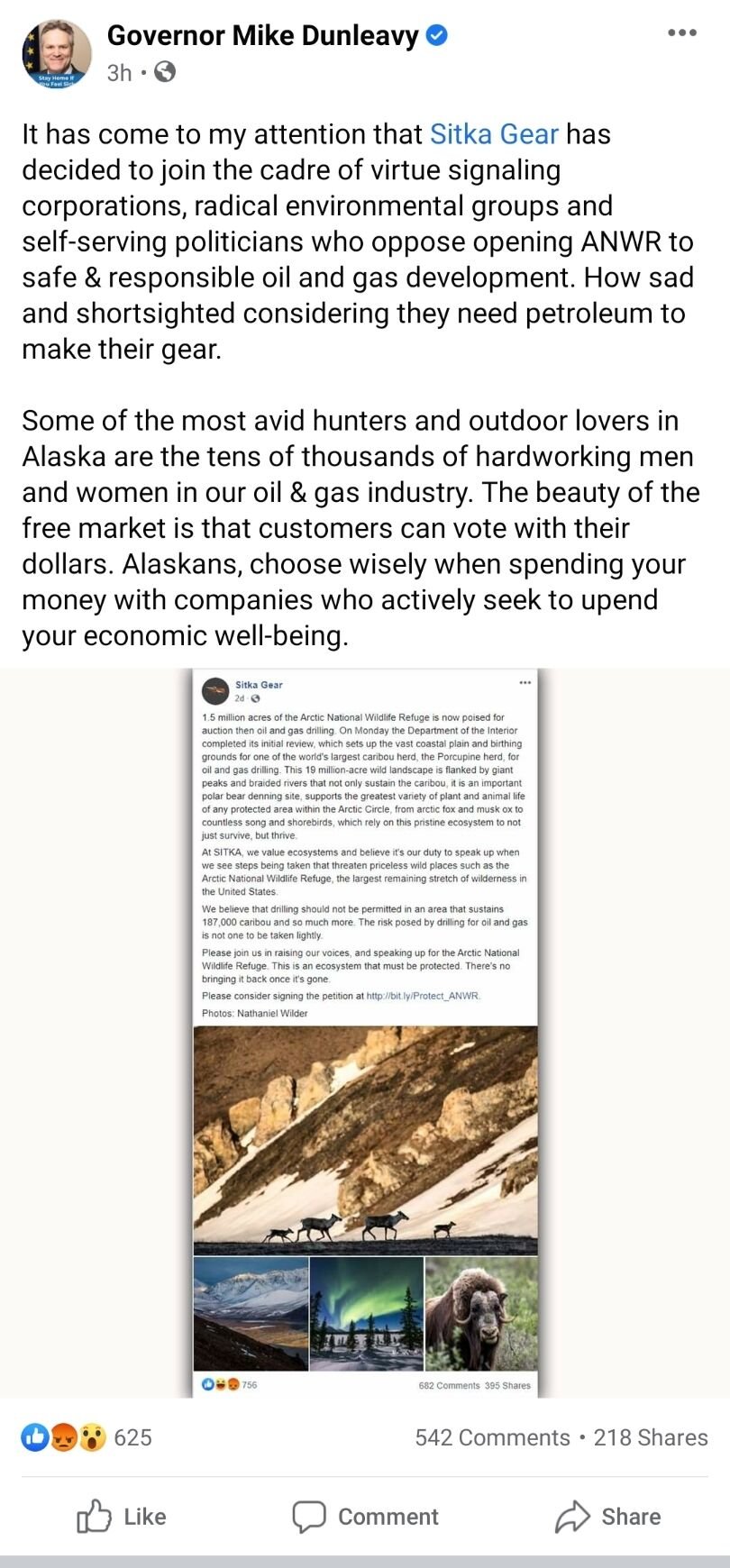In this image, the layout is indicative of a Facebook post. At the top of the post, the author is identified as Governor Mike Dunleavy, verified by a blue checkmark next to his name. In the post, Governor Dunleavy expresses his concern and criticism over Sitka Gear’s stance on opposing the opening of the Arctic National Wildlife Refuge (ANWR) for oil and gas development. He labels Sitka Gear as part of a group of "virtue signaling corporations, radical environmental groups, and self-serving politicians."

Governor Dunleavy argues that the opposition is "sad and short-sighted," highlighting the irony that Sitka Gear, which manufactures products for hunters and outdoor enthusiasts, relies on petroleum for production. He emphasizes that many avid hunters and outdoor lovers in Alaska work in the oil and gas industry and suggests that they are integral to the state’s economy.

The governor advocates for the power of the free market, encouraging Alaskans to consider how their spending choices impact their economic well-being. He underscores the importance of supporting companies that align with their economic interests.

At the post's bottom, engagement metrics show approximately 625 reactions, 542 comments, and 218 shares, indicating substantial interaction within three hours since it was posted, as per the timestamp. Navigation buttons for liking, commenting, and sharing the post are visible, marking it as a standard Facebook post format.